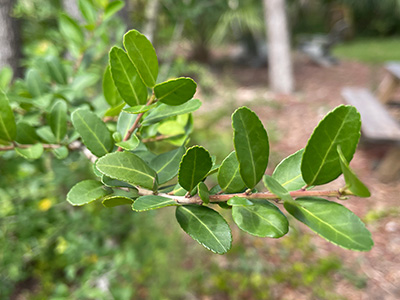This is a close-up photograph of a plant branch, prominently featuring green, oval-shaped leaves along a reddish-brown stem. The stem runs horizontally from the right side of the image to the left and bends slightly towards the camera in the middle. The lush leaves, with some lighter green veins, are in sharp focus at the front, gradually fading into blur at the back. 

The background is softly blurred with a bokeh effect, highlighting various elements indicative of a park setting. To the left is another out-of-focus bush, and to the right, you can see parts of a wooden picnic table and bench. The ground is brown and leads up to the trunk of a tree, which extends to the top of the picture, emphasizing the height of the camera view. The overall scene suggests a serene outdoor environment, devoid of people, focusing purely on the natural elements.